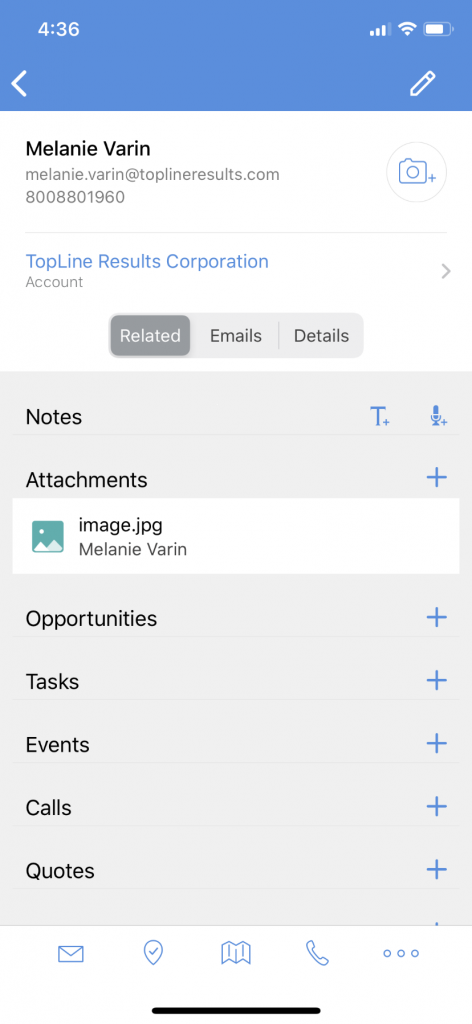A detailed and refined caption for the image could be:

"A screenshot of a smartphone interface displays various pieces of information. The time at the top reads 4:36, enclosed within a blue border. In the same bar, three out of four signal bars are shown, along with a full Wi-Fi connection and a battery at approximately 75% capacity. Below this are two icons: a left-facing arrow on the left and a pencil icon on the right. 

The screen prominently displays the name "Melanie Varon" and her email "melanievaron@toplineresults.com". An oval-shaped icon containing a camera is visible next to the phone number "800-880-1960". Below this, the text "Top Line Results Corporation Account" is shown in blue. 

Three buttons are present underneath: a dark gray one labeled "Related", and two light gray ones labeled "Email" and "Details", respectively. Further down, a gray box contains categories labeled "Notes Attachments image.jpg", "Melanie Varon Opportunity Tasks Events Calls and Quotes".